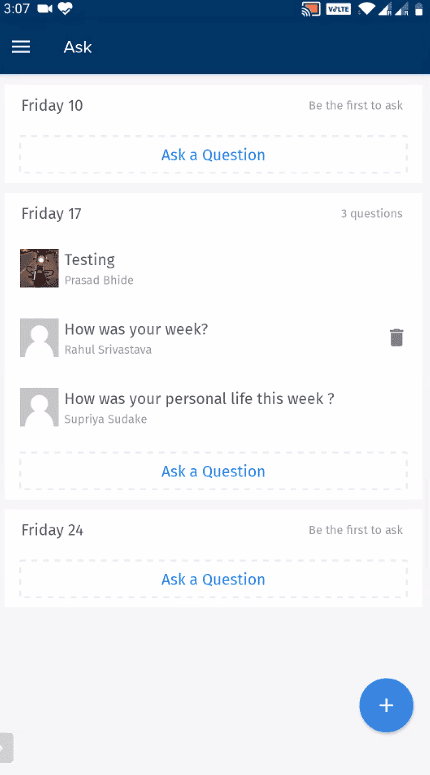This screenshot, captured on a mobile phone at 3:07 PM on a cloudy day, shows the interface of an app. At the top of the screen, the status bar indicates an average cellular signal strength and an unclear battery level. The header section of the app displays "Friday 10" with the prompt "Be the first to ask," followed by a blue "Ask a question" box.

Below this, the app lists the date "Friday 17" accompanied by three existing questions: "Testing for us," "How was your week?" by Rahul Srivastava, and "How is your personal life this week?" by Shoaib Saddique. Each question is marked with a blue highlighted text for adding new queries. Further down, for the date "Friday 24," the prompt "Be the first to ask" reappears alongside another "Ask a question" box in blue.

The interface concludes with a prominent blue circle containing a plus sign situated at the bottom right corner, suggesting an option to add new content or actions.